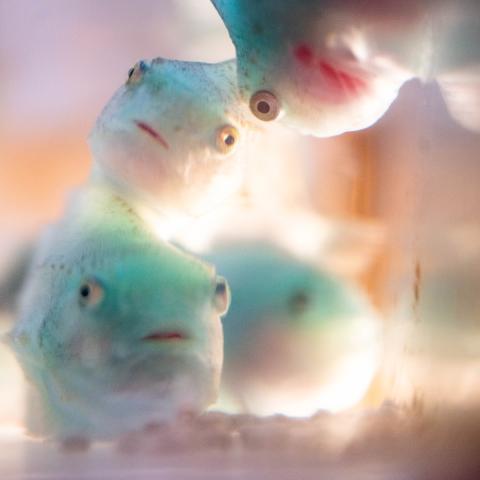The image showcases four distinct emerald-turquoise, translucent Cyclopterus fish within an aquarium-like container. The scene is divided, with two fish resting on a white surface near the bottom of the image and the other two appearing to float or swim at the top. The fish are notable for their wide-set, circular eyes with prominent black pupils contrasted against large eye whites. Their bodies display a unique transparency allowing light to refract through their skin, giving a glimpse of internal nuances. The fish have small mouths, and one of them is partially open, revealing a hint of red inside. The background features out-of-focus elements, including some pink, light orange, and faint purple tones, and possibly marbles or decorative elements at the bottom. Additionally, a mirror on the right side of the image reflects parts of the scene, enhancing the aquarium's depth and abstract aesthetic. Some fish have visible gills, spots, and fins, with blunt noses and slightly raised backs capturing the diverse anatomical features of these unique fish.